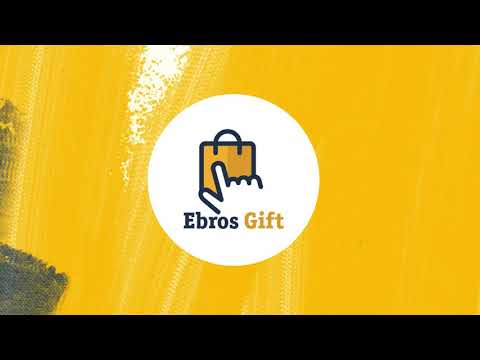The image features an advertisement or logo centered on a bright gold-yellow background, punctuated with shininess on the left-hand side and some lighter yellow streaks throughout. The top and bottom sections of the image are bordered with black horizontal lines, and there's a gray smear in the lower left corner. Dominating the center of the image is a white circle containing the detailed outline of a hand with the thumb and forefinger outstretched, pressing on what appears to be a dark yellow shopping bag outlined in black with a black handle. Beneath the hand, the text "EBROS" is written in black, followed by "GIFT" in yellow. The overall design suggests a polished advertisement possibly for a shopping or gift-related service.